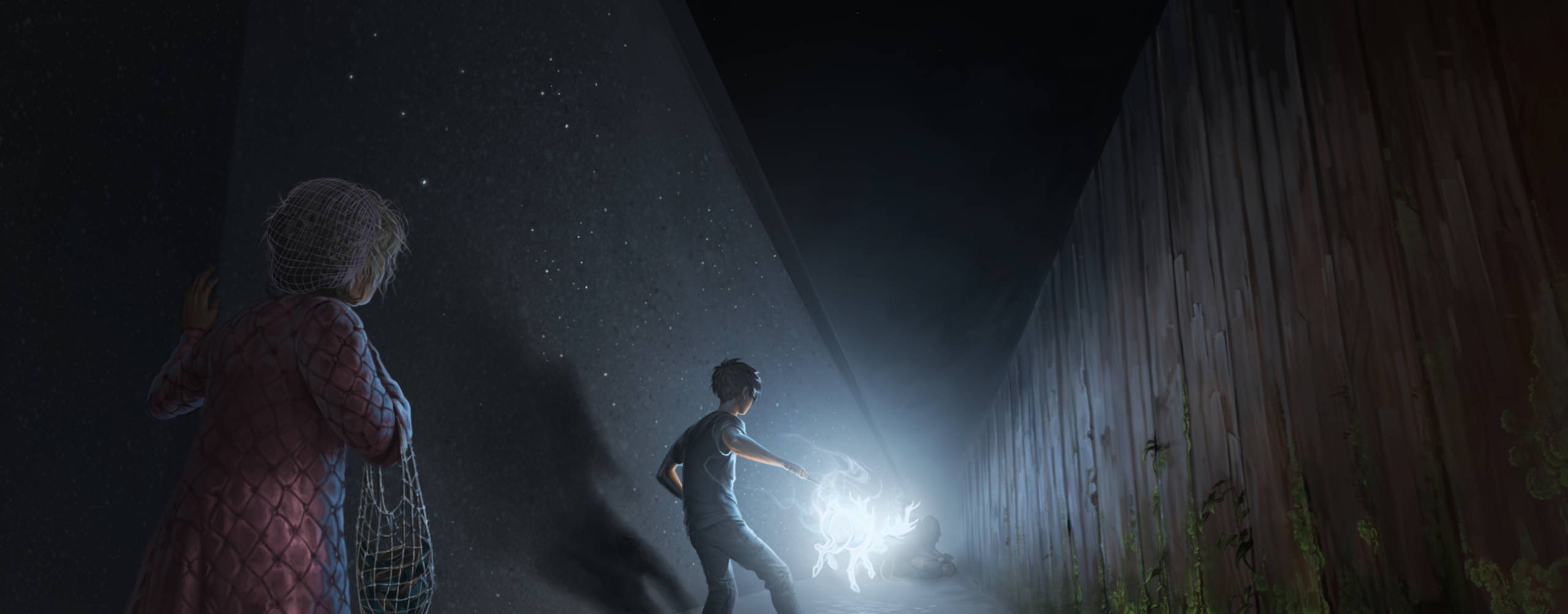The image appears to be a vivid digital painting or animated drawing depicting a supernatural scene in a dark hallway. In the foreground, a young boy around 10 years old, dressed in a blue short-sleeve shirt and jeans, stands at the center. He is gazing at a bright, white spectral light or flame-like figure right in front of him. The hallway is defined by two distinct walls on either side; the right wall resembles a wooden fence, while the left wall appears to be a harder, concrete-like surface with white specks. In the bottom left corner, more towards the edge, an older woman with gray hair pulled up, dressed in a long purple and blue dress and holding a mesh net purse, looks on towards the boy. The overall setting exudes an eerie, magical atmosphere with colors including bright white, black, sleek reddish tones, gray, beige, and tan.